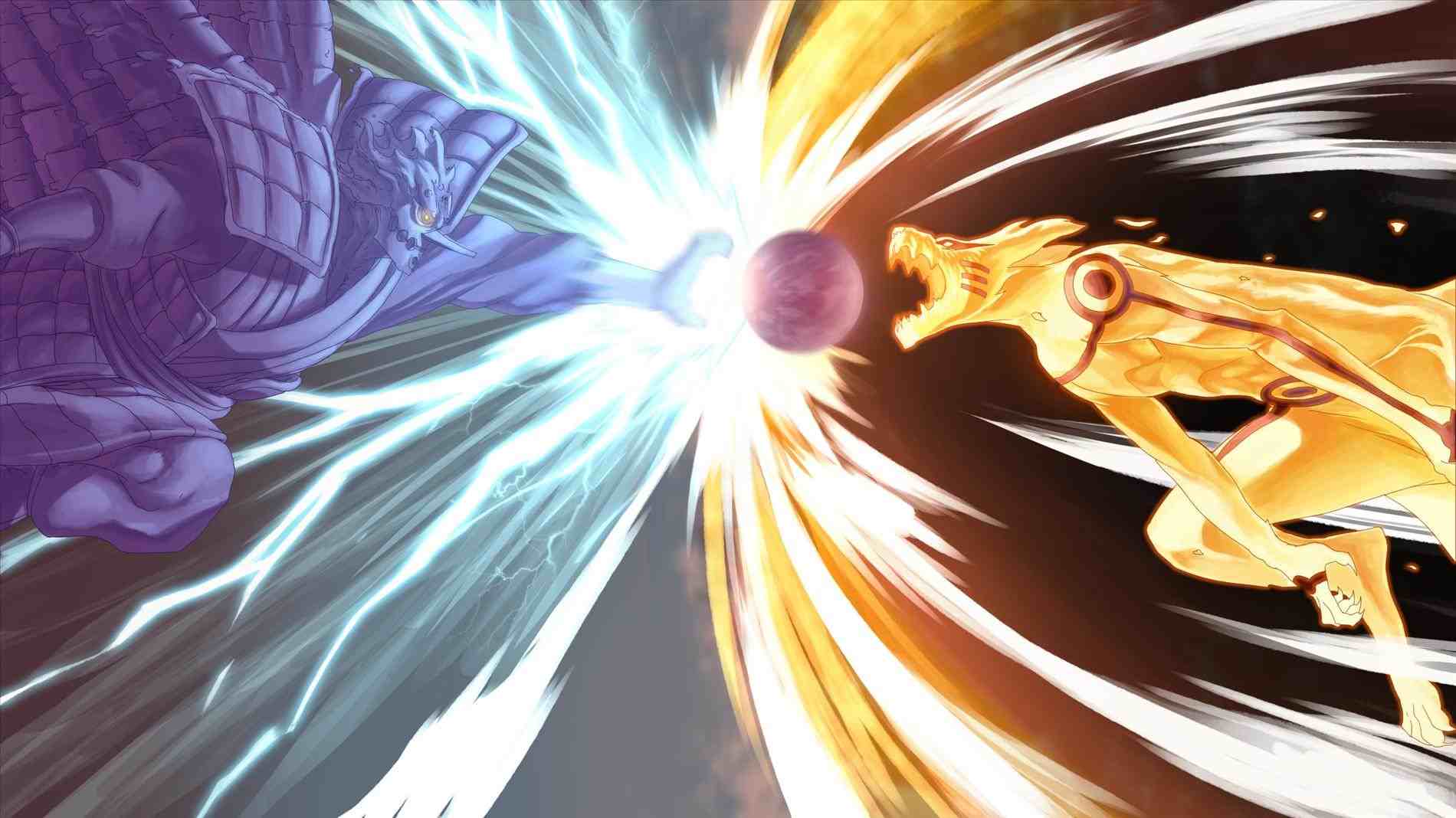The image displays a highly detailed, animated-style artwork showcasing a scene with two mythical creatures against a black backdrop. On the right side, there is an orange creature with a lion-like or wolf-like humanoid body, lunging forward with its mouth open, seemingly trying to bite a pink or red ball in the center. This creature features large fangs, a human-like body with some animalistic traits, and has a red target-like pattern with lines emanating from it, suggesting rapid movement and force. On the left side, a wicked-looking purple character with a sharp, pointed nose, wild purple hair, and glowing yellow eyes is depicted. This character is adorned in heavy armor, possibly a thick coat with a cape and a hat, and is reaching out with its left hand towards the same ball. There are light blue lightning effects around it, adding to the dynamic tension of the scene. Both characters are depicted in action, converging on the ball in the middle of the image, with blue lightning and white velocity lines accentuating the sense of movement and urgency.